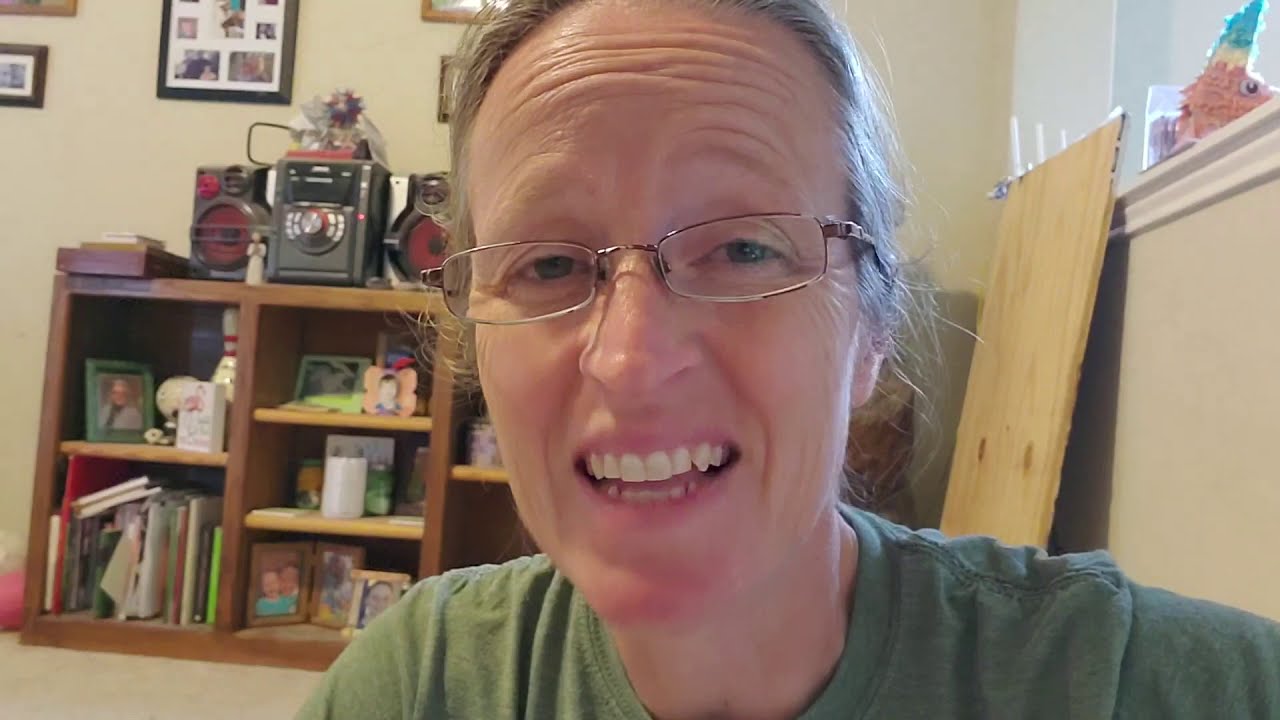In this photograph, an older woman with slightly whitening hair is centered prominently, making a slightly disgusted face, wrinkling her forehead and with her mouth open, revealing her top and a bit of bottom teeth. She wears small, wire-rimmed glasses with lenses wider than they are tall, and a dark green T-shirt. Her hair is pulled back, and she sits against a beige wall, possibly on a tan carpet. To her left, there is a shelf filled with various items including books, numerous picture frames, and a stereo system with black outer speakers and red inner parts. Additional picture frames are mounted on the wall above the shelf. To her right, under a windowsill, there is a large piece of plywood leaning against the wall. Resting on the windowsill is the colorful head of what appears to be a piñata, highlighted by sunlight. The room has a somewhat cluttered yet personal feel, filled with cherished photos and possessions.